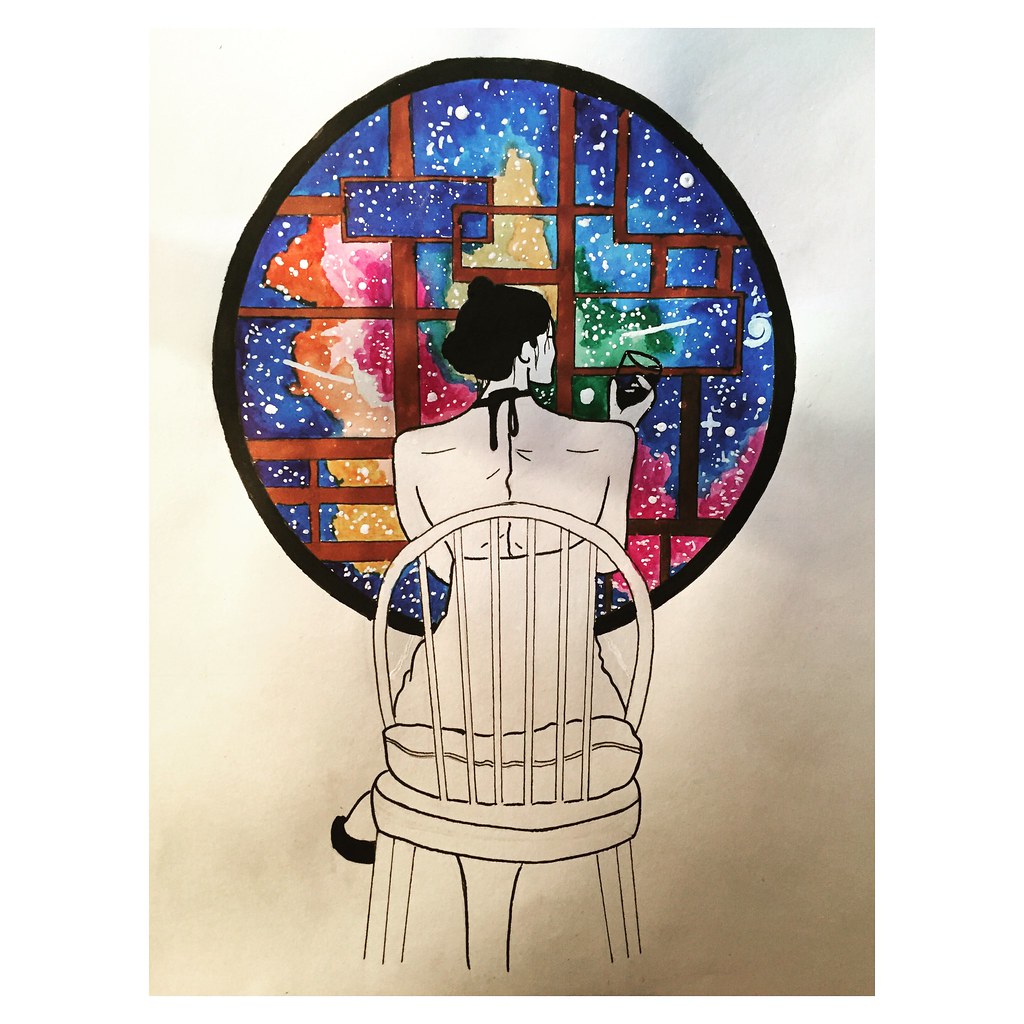This is a detailed illustration of a woman sitting in a circular, cushioned chair with her back turned towards the viewer. She is wearing a backless nightgown or dress, tied into a bow at the nape of her neck. Her hair, which is black and neatly tied up, complements her black shoes or slippers. The woman is depicted holding a glass, seemingly filled with a dark liquid, in her right hand. 

The setting features a round window or multicolored painting in front of her, characterized by a complex pattern of lines and shapes, both square and rectangular, with no curves. The scene outside or depicted within the window resembles a starscape, with a predominantly blue background adorned by an array of colors—green, yellow, red, orange, and pink—suggestive of a nebula, all speckled with white stars.

The woman's chair and cushion appear white, though the photographic nature of the image imparts a beige hue to them. The entire illustration is in outline form, void of color, lying against a beige background that shifts to a darker shade towards the bottom. The overall composition captures the serene ambiance of the woman gazing thoughtfully at the vibrant, cosmic scene before her.